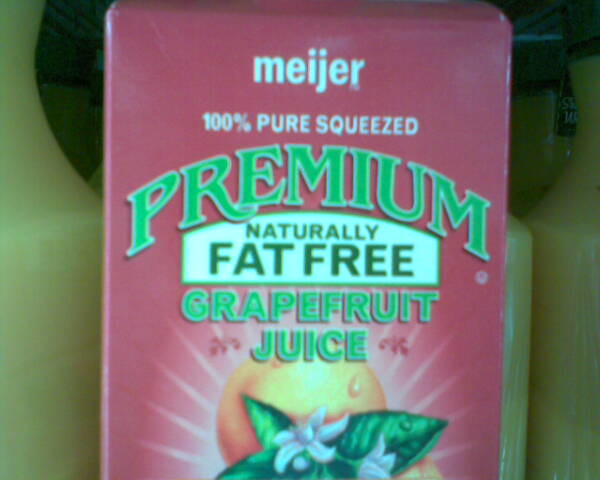The image features a vibrant and colorful design primarily divided into distinct sections: 

On both the left and right sides, rich green elements frame the composition, giving a sense of freshness and vitality. Dominating the center of the image is a prominent red box. Inscribed across this box in bold white text are the words "Measure and Algebra," suggesting a precise and scientific approach.

The image further details a message indicating "100% Squeeze," possibly referring to pure, freshly-squeezed juice. Just below, green text stretches across an orange banner, indicating something premium. Underneath this banner is another section with pink text that proudly states "Naturally Fat-Free."

Labeled as "Grapefruit Juice" in white text, the product is visually emphasized by a large, eye-catching grapefruit illustration. This grapefruit is depicted with realistic droplets of moisture, surrounded by lush green leaves and a delicate white flower, enhancing the freshness appeal. Additionally, sparkles and light reflections are artistically rendered around the grapefruit, adding a touch of vibrancy and making it appear even more enticing.

Despite the visually appealing and lively composition, the image itself is slightly grainy, suggesting a lower image quality.